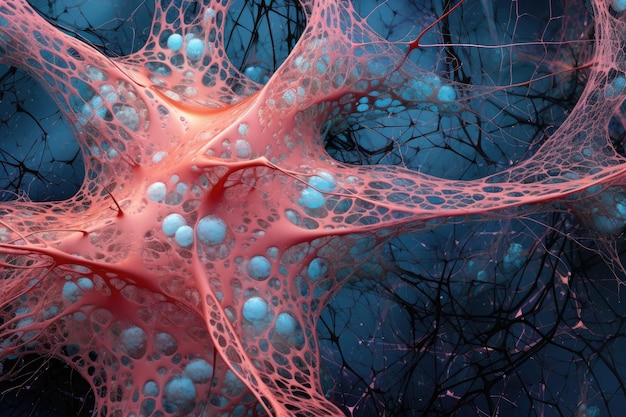The image depicts a detailed 3D rendering of a neuron within the brain, centrally positioned on the left side. The neuron, a web-like structure in varying shades of pink and orange, features an intricate series of holes and stretches outward into a star-like shape. Dotting the neuron both within and surrounding it are numerous blue orbs, which suggest cellular activity. Surrounding this focal point, the background transitions from dark blue in the lower sections to a lighter blue towards the top and left, evoking a watery environment. Dark, black crisscrossing branches silhouette across the background, with a few closer ones rendered in red or pink hues, extending further into the scene and connecting with more blue orbs in the distance. The depiction captures the essence of a neural network, stretching towards the top right corner, providing a mesmerizing blend of scientific representation and artistic abstraction.